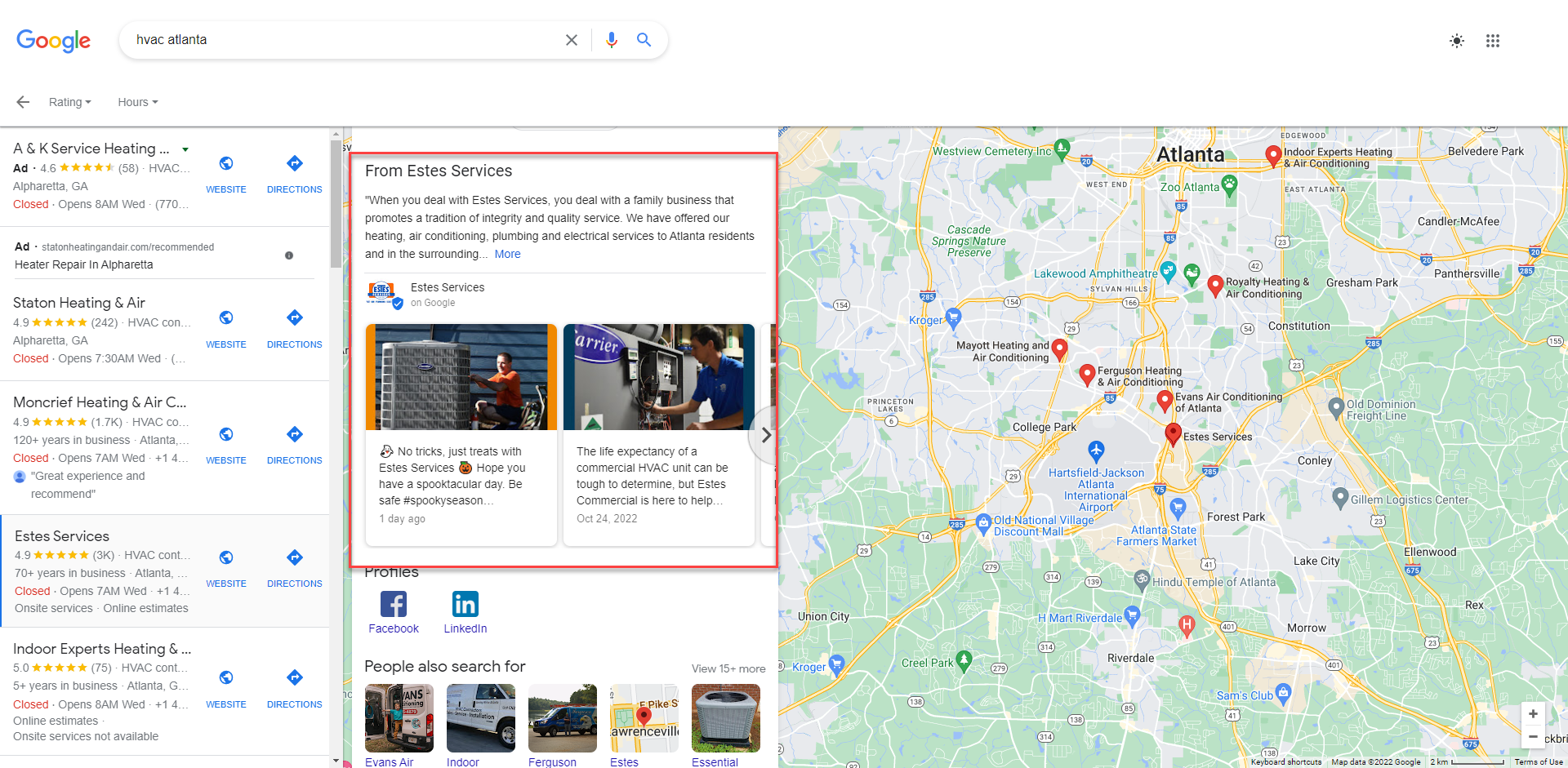This detailed screenshot captures a Google Maps interface on a digital device—potentially a desktop, laptop, smartphone, or tablet. The map occupies the right-hand side of the screen, adorned with numerous red and green pins marking various locations. Blue highway signs with shields and a red top band, along with a network of roads, some of which are colored orange, add layers of detail to the map. The image also showcases areas in gray, green fields, and blue waterways.

At the top URL bar, the search term "HVAC Atlanta" is visible. On the left-hand side of the screen, the Google logo appears in its iconic colors: a blue "G," followed by a red "o," a yellow "o," a blue "g," a green "l," and a red "e." Beneath the logo are options marked by a red arrow and labeled "Rating" and "Hours," each with a drop-down menu.

Listed below this section are multiple HVAC service businesses, each accompanied by ratings, reviews, and additional details:

1. **H&K Service Heating**:
   - Rating: 4.6 out of 5 stars (58 reviews)
   - Status: "Ad" in bold black text
   - Location: Atlanta, Georgia
   - Operational Status: Closed (in red); Opens at 8 AM on Wednesday
   - Contact: Partial phone number starts with (770)
   - Additional Info: Website and directions available

2. **Heater Repair in Alpharetta**:
   - Status: "Ad"
   - Location: Alpharetta, Georgia

3. **Station Heating and Air**:
   - Rating: 4.9 out of 5 stars (242 reviews)
   - Location: Alpharetta, Georgia
   - Operational Status: Closed (in red); Opens at 7:30 AM on Wednesday
   - Additional Info: Website and directions available

4. **Monarch Heating and Air**:
   - Rating: 4.9 out of 5 stars (1.7K reviews)
   - Operational Status: Closed (in red); Opens at 7 AM on Wednesday
   - Additional Info: 120 years in business, partial phone number starts with +1 4, website, directions, and a partial review indicating a "great experience and recommend."

5. **Estes Services**:
   - Rating: 4.9 out of 5 stars (3.3K reviews)
   - Operational Status: Closed (in red); Opens at 7 AM on Wednesday
   - Additional Info: 70 years in business, partial phone number starts with +1 4, website, directions, and offers on-site services and online estimates

6. **Indoor Experts Heating**:
   - Rating: 5.0 out of 5 stars (75 reviews)
   - Operational Status: Closed (in red); Opens at 8 AM on Wednesday
   - Additional Info: 5+ years in business, partial phone number starts with +1 1, website, online estimates, and services not available

This comprehensive caption provides an in-depth description of the Google Maps search results for HVAC services in Atlanta, complete with business information, ratings, operational hours, and additional service details.